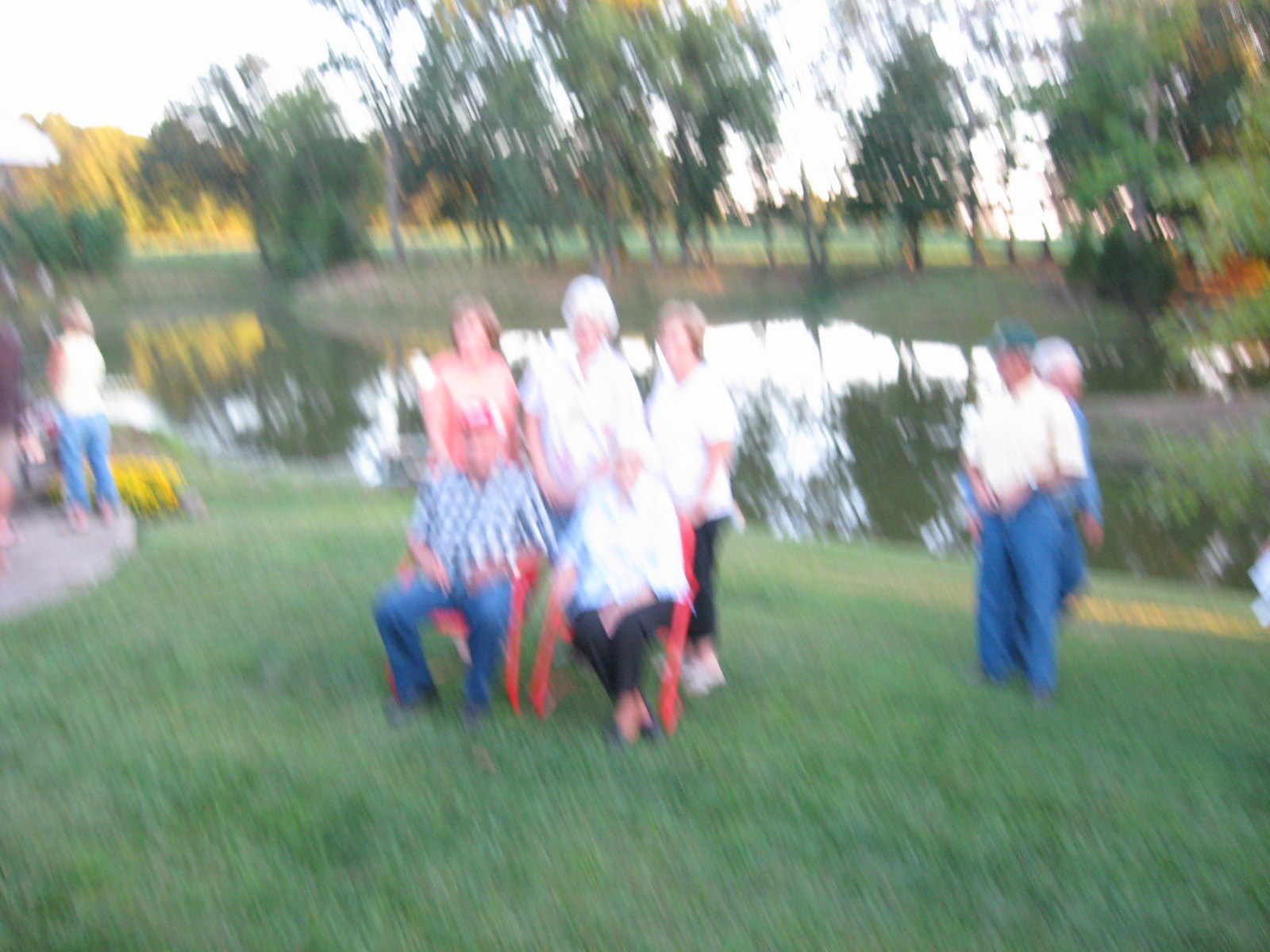This very blurry photograph captures a family reunion or friends and family gathering in a well-maintained park or backyard setting. Central in the image are an elderly couple seated on red plastic chairs—the man is dressed in a blue and white checkered shirt, blue jeans, and a red and white baseball cap, while the woman wears black pants and a white shirt, with white hair. Standing behind them are three women: two with light brown hair and white shirts, and one with white hair in an orange shirt. To the right, there are two men in blue jeans—a third man in a green baseball cap and pale yellow shirt, and another man who is dressed in blue with white hair. Off to the left, there's a woman in blue jeans with her back turned, wearing a white top. The group is gathered on a grassy lawn in front of a pond or lake, with more grass, fields, and trees on the other side. The sky, almost white, suggests a bright, sunny day.